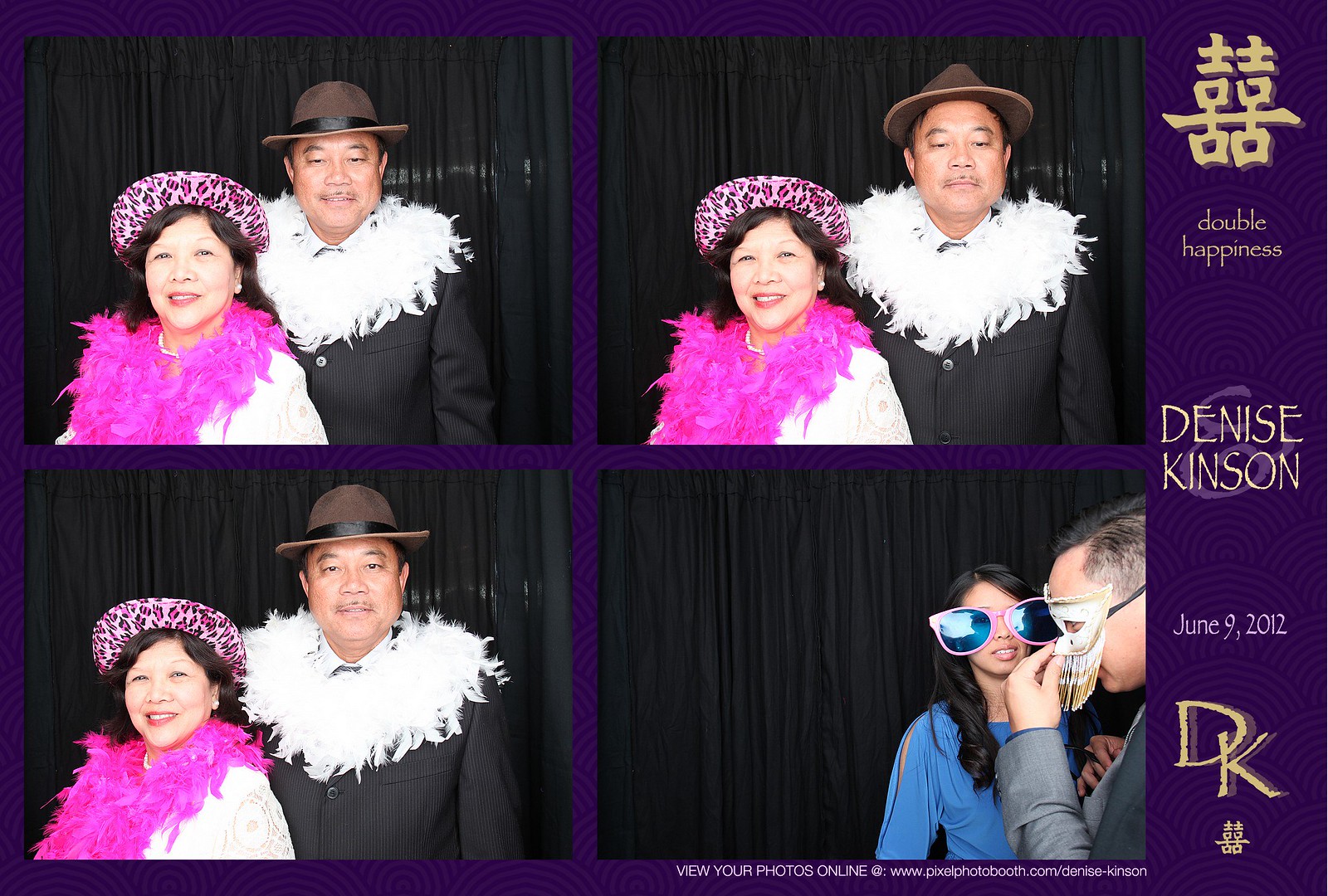The image depicts a series of four photo booth pictures, captured at what appears to be a wedding event on June 9th, 2012, for Denise Kinson. The photos are arranged in a 2x2 grid on a purple background, with a vertical strip on the right featuring gold Asian lettering and the words "double happiness," along with the name "Denise Kinson" and the initials "DK." At the bottom, there's a message directing viewers to "view your photos online at www.pixelfotobooth.com/DeniseKinson."

In the first three photos, a man and a woman, both appearing to be in their late 40s or mid-50s and of Asian descent, are the focal point. The man stands behind the woman and is dressed in a black suit with a brown hat featuring a black band. He accessorizes with a large white feathered boa draped over his shoulders. The woman stands in front, wearing a white shirt paired with a pink leopard print hat and a pink feathered boa. In these images, they alternate between smiling directly at the camera and more candid expressions. 

The fourth photo, located in the bottom right corner, captures a different pair of individuals, seemingly younger. The young woman, also of Asian descent, sports long curled black hair, a long-sleeved blue blouse, and oversized pink sunglasses. Accompanying her is a man partially visible from the left, wearing a gray suit and adjusting a brown fringe mask, likely in the midst of entering the booth.

Overall, the photo series captures the joyful and playful atmosphere of a wedding photo booth, enhanced by the use of whimsical props and expressive poses.